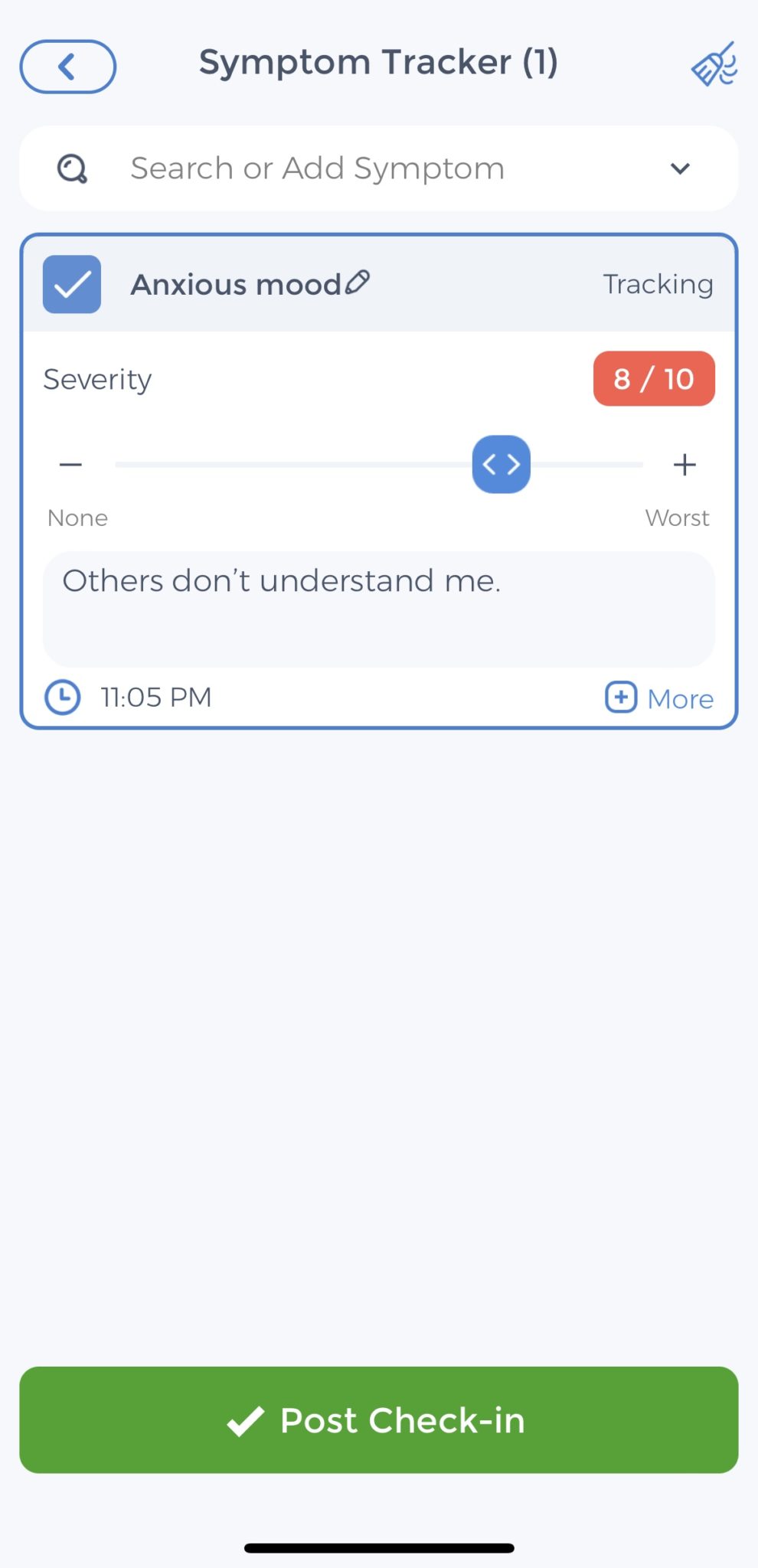The image depicts a mobile screenshot, likely from an Apple device, given the distinctive line at the bottom used to minimize the app. The app shown is a symptom tracker.

### Detailed Caption:
The screenshot displays the interface of a symptom tracking app on a mobile device. At the top, there is a rectangular icon with curved sides and a left-facing arrow, indicating a navigation or back button, labeled "Symptom Tracker (1)." Adjacent to it on the right is a small icon of a blue and white broom, symbolizing a cleaning or clear function.

Below this is a search box with a magnifying glass icon, labeled "Search or add symptom," accompanied by a dropdown menu. The user’s current mood is indicated with a blue checkmark and described as "anxious." Next to this, a severity indicator is displayed within a red square, rating their anxiety at "8 out of 10."

The severity can be adjusted using a drag bar—depicted as a blue rounded square with white arrows—ranging from "none" to "worst." Underneath this bar, there's a text box where the user has written, "Others don't understand me." The timestamp for this entry is 11:05 PM. An option to "Add More" is available below the text box.

At the very bottom is a green rectangle with a white checkmark and the words "Post Check-In," suggesting a button to submit or record the current entry. This app appears to be designed to help track and manage emotional and physical symptoms.